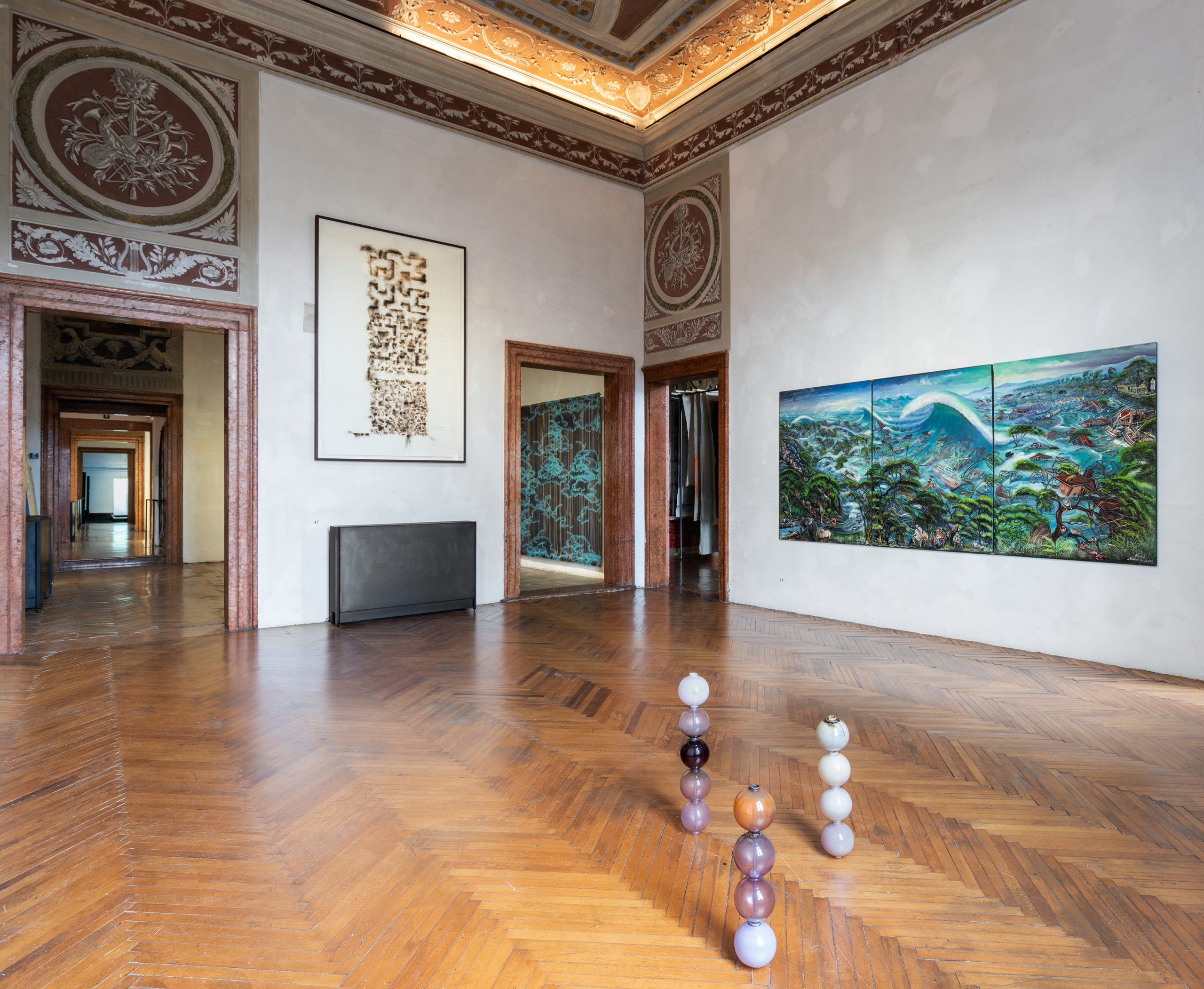The photograph depicts an expansive interior space, likely an art gallery or museum with tall, vaulted ceilings adorned with intricate plaster friezes and brocade-like decorations in metallic and golden tones. The wooden floor, meticulously maintained and arranged in a herringbone pattern, stretches across the room. The focal point of the room is three stacked sculptures of spherical orbs made of various materials and colors, including white, purple, orange, black, and gray, each supported by metal rods—with one stack containing five spheres and the other two containing four.

The room features a series of wall-mounted artworks, which include a large three-panel painting with a nature scene depicting water and trees, likely in an Asian style. This painting occupies much of the right wall. Opposite it, there is a doorway leading to what appears to be a closet or a space with hanging clothes. Another significant artistic detail includes a teal and brown painting with various geometric shapes, placed between doorways on the left wall. Additionally, the space connects to other rooms via several doorways, lining a hallway that extends into the distance.

Above each doorway, elaborate engravings in red, blue, and gold add to the ornate condition of the room, reminiscent of traditional Asian architectural elements. The sunlight streaming down from a skylight enhances the ethereal atmosphere of the gallery, highlighting both the sculptures and the artworks on the walls. The overall impression is one of serene emptiness, with the sculptures and the artworks serving as the primary points of focus.